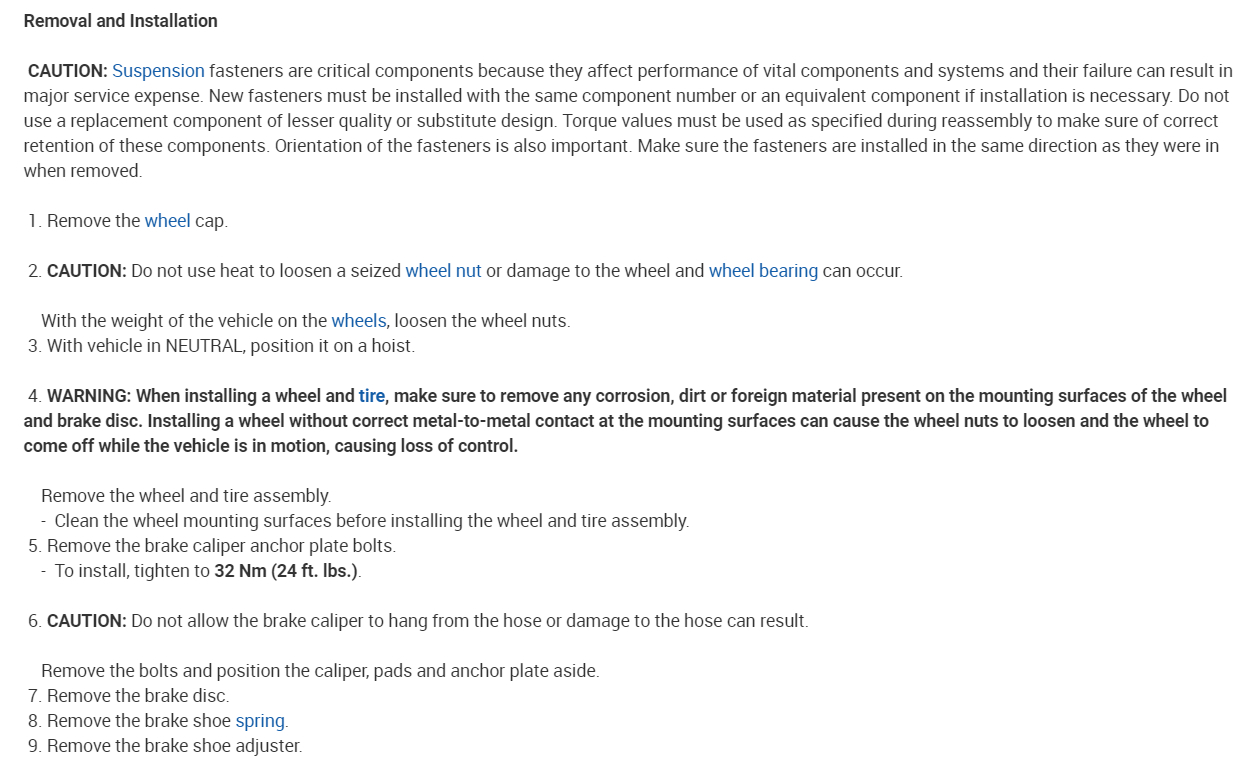**Detailed Caption:**

**Warning/Caution Text Documentation for Suspension Maintenance**

The image showcases a detailed instruction manual page, focusing on the removal and installation of suspension components. The title "Removal and Installation" is prominently displayed in bold black letters, followed by a bold uppercase "CAUTION". The word "Suspension" is highlighted in blue text, emphasizing its significance.

The caution text warns that suspension fasteners are crucial because they impact the performance of vital components and systems. Failure of these components can lead to significant service expenses. It is imperative to install new fasteners with the same component number or an equivalent component when necessary. The caution stresses not to use replacement components of lesser quality or substitute designs, and to adhere to specified torque values during reassembly.

Below the caution information, the image lists steps numbered from one to nine for the removal and installation process:

1. **Remove the wheel cap.**
2. **CAUTION**: Do not use heat to loosen the wheel nut as it can damage the wheel bearing.
3. With the vehicle in neutral, position it on a hoist.
4. **CAUTION**: When installing the wheel and tire, ensure the removal of any corrosion or dirt.
5. Remove the brake caliper anchor plate bolts.
6. **CAUTION**: Do not allow the brake caliper to hang from the hose as it can damage the hose.
7. Remove the brake disc.
8. Remove the brake shoe spring.
9. Remove the brake shoe adjuster system.

Each step is detailed and precautions are clearly highlighted to ensure proper and safe maintenance procedures.